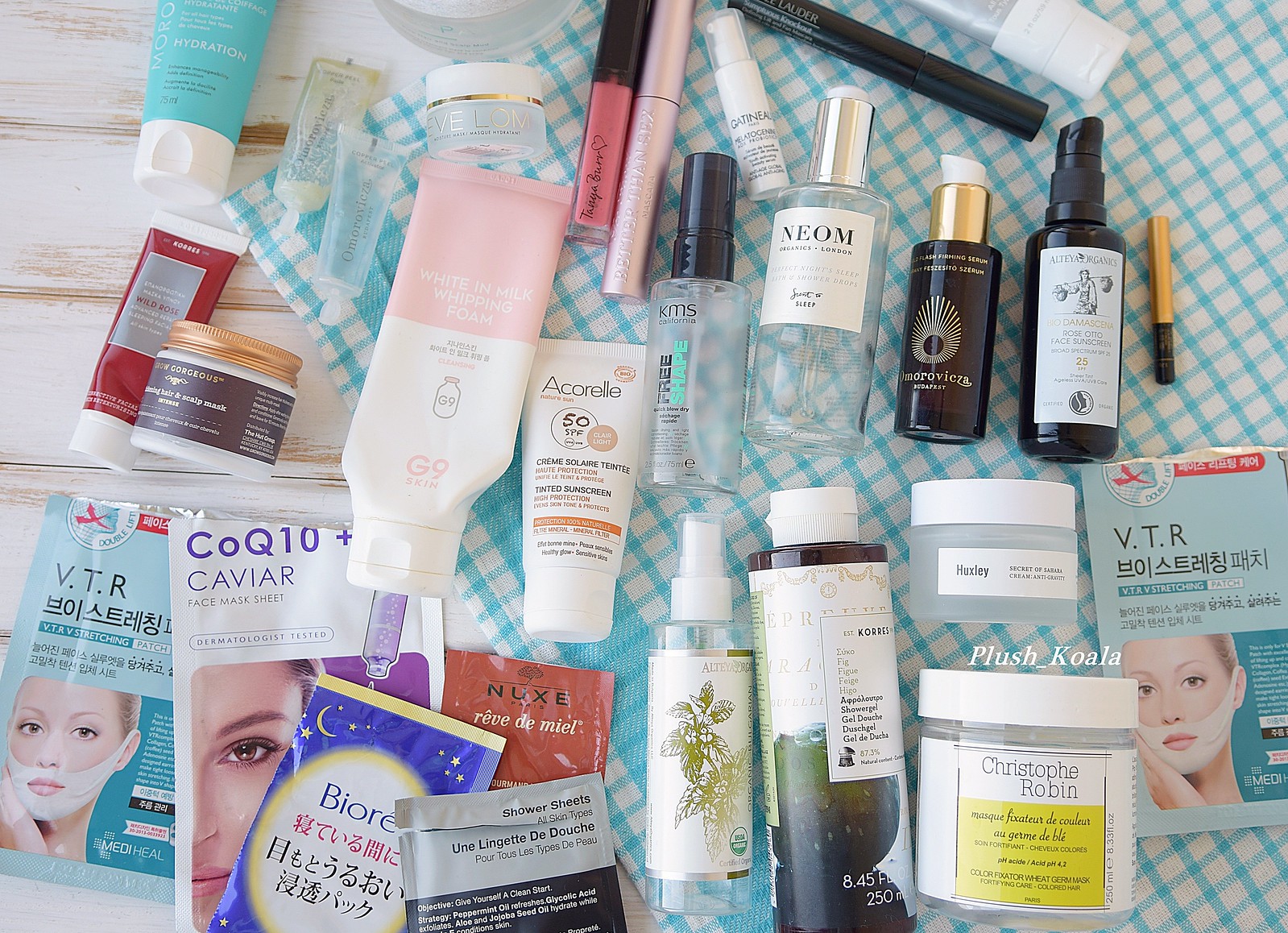In this top-down image, we observe a curated arrangement of various makeup and skincare products alongside an assortment of magazines. 

On the bottom left, there is a light blue magazine labeled "VTR," featuring text in a non-English script and an image of a woman with foam on her face against a blue background. Adjacent to this on the right is another magazine titled "COQ10+," highlighting the word "caviar" in purple with a female model and a purple backdrop.

To the right of this magazine, a blue book with a distinctive yellow and white circular design on the cover is visible. Below this book lies a brown book, and above it is a gray and black book. Interspersed among these publications are a couple of small bottles with white caps—one positioned at the bottom and one at the top.

On the far right, there's a dark brown and white bottle with a wide container and white cap. Directly above it, another bottle with similar styling can be seen, and next to both, another VTR magazine appears.

At the top of the arrangement, a small brown and black utensil is placed. To its left sits a black spray bottle. Continuing leftward, there is a black bottle with a gold cap, followed by a clear bottle with a white label and a silver or gold cap. Further left, a clear bottle with a black cap is located.

Below this sequence resides a white bottle with the name "XRL" inscribed on it. Adjacent to the left is a half pink, half white bottle with a bottom cap, and next to it, a compact jar featuring a chrome bronze lid. Left of this jar, a small red bottle is spotted with additional makeup products arranged above it. A small blue bottle with a white cap occupies the top left corner of the scene.

The backdrop beneath the objects on the left consists of white wooden planks, whereas to the right, the background transitions to a blue and white small checkered cloth, creating a vivid contrast.